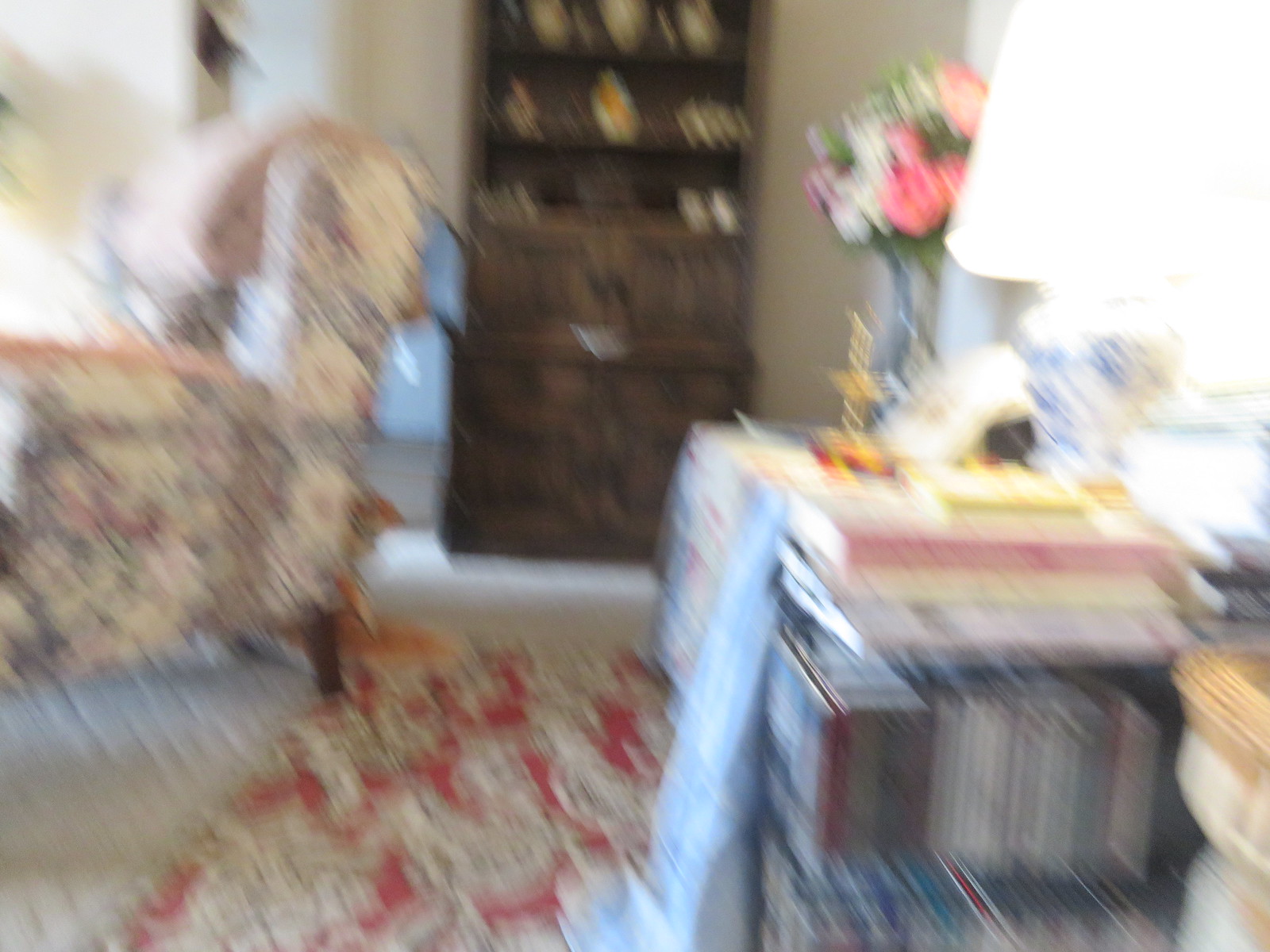This image showcases a cozy, traditionally decorated living room, likely owned by an elderly woman, as suggested by the vintage-style furniture and decor. On the left side of the room, a white armchair adorned with blue floral patterns catches the eye, though its details are slightly obscured by a pervasive motion blur. In front of the chair, there appears to be a red carpet with intricate white designs. A small table sits a bit closer to the camera, topped with a vibrant arrangement of red and white flowers, accompanied by green leaves, a golden candlestick holder, and a white pot featuring blue designs. 

This table, positioned under the soft light of a white lampshade, adds a warm, welcoming glow to the room. At the back, a dark brown cabinet, filled with plates and various vases, stands against the wall, showcasing an array of delicate ornaments and adding to the room's classic charm. The combination of these elements creates a warm and nostalgic atmosphere, characteristic of an older generation's home.